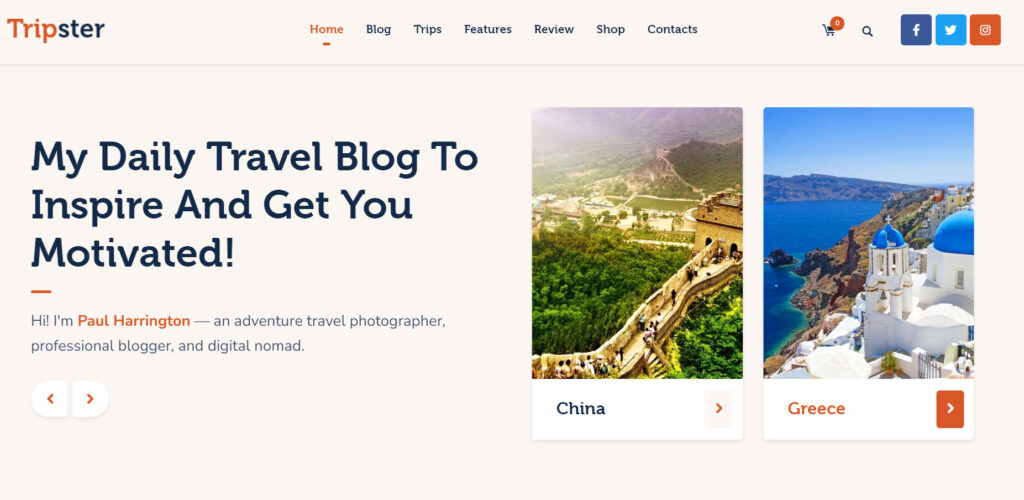In the upper left-hand corner of the image, we see the website header for Tripster. The header prominently features the word "Tripster" with "Trip" in an orange-reddish font and "ster" in black. This header runs horizontally across the top in a menu bar, which houses the main navigation options centrally located on the screen: Home, Blog, Trips, Features, Review, and Contacts. To the right of these options, there is a shopping cart icon indicating six items, followed by a search magnifying glass symbol. Adjacent to this are three social media buttons, sequentially representing Facebook, Twitter, and Instagram.

Beneath the navigation menu, a large, bold black font announces, "My Daily Travel Blog to Inspire and Get You Motivated." Directly below this title, a smaller font introduces, "Hi, I'm Paul Harrington, an adventure travel photographer, professional blogger, and digital nomad."

On the right-hand side of the screen, adding visual interest, are two picturesque images: one of scenic landscapes in China and the other of stunning vistas in Greece.